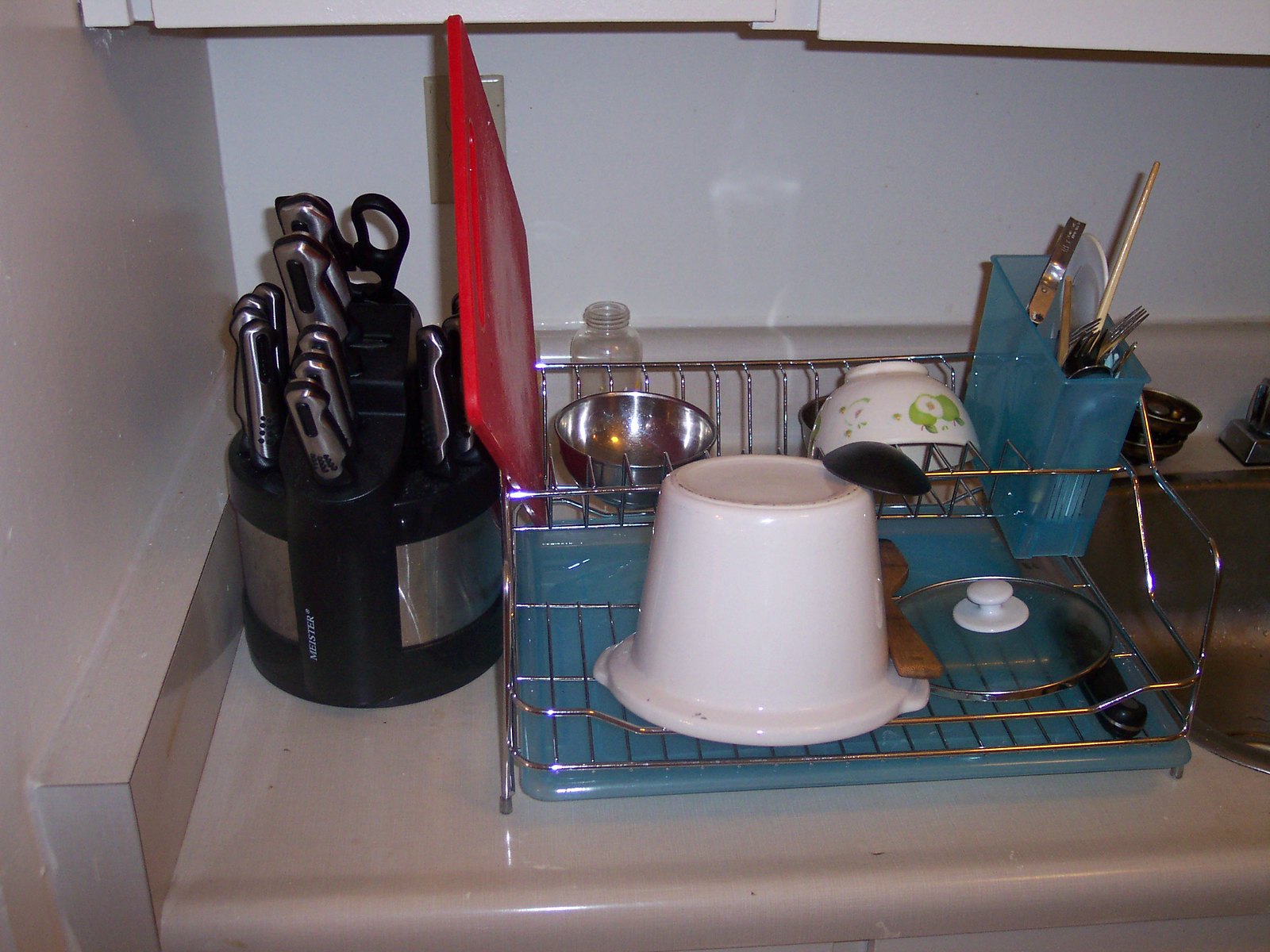This photograph captures a compact kitchen workspace, showcasing efficient use of a limited area. The countertop, made of green Formica, measures approximately two and a half square feet and sits adjacent to a stainless steel sink. A black cylindrical knife block occupies part of the counter, housing an assortment of knives with silver and black handles, including several steak knives, paring knives, a large meat or butcher knife, and a pair of kitchen scissors, all neatly slotted.

Next to the knife block, there's a dish drying rack filled with various kitchen essentials. Among them is a well-used red plastic cutting board, a metal mixing bowl, a steel bowl, and a crock. Also present is a lid with a plastic button handle, a rice bowl, and various utensils stored in a plastic holder with holes, resembling a colander. This detailed setup emphasizes the kitchen's functionality despite its small size.